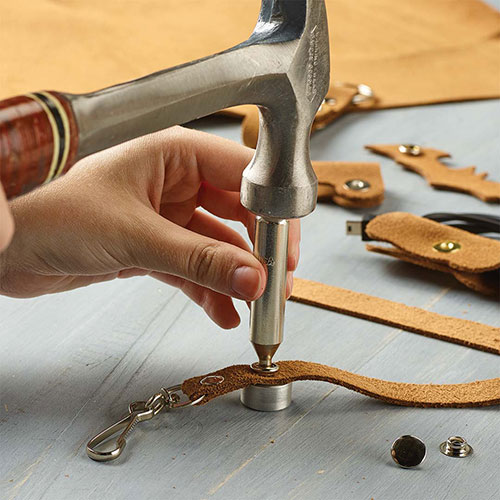In a brightly lit workspace, a close-up image captures a woman's hand meticulously crafting a leather dog leash. She wields a regular hammer with a brown wooden handle and a silver metal head to punch rivets through the tan-colored, rough, and suede-like leather. The leather strip, adorned with a decorative tortoise shell button snap, is attached to a silver latch and hook, reminiscent of a lanyard. The scene is set against a gray table, with other assorted leather pieces, including some with rivets, scattered in the background. She holds a specialized punch tool, guiding the rivet precisely into place, showcasing the detailed craftsmanship of leatherworking.